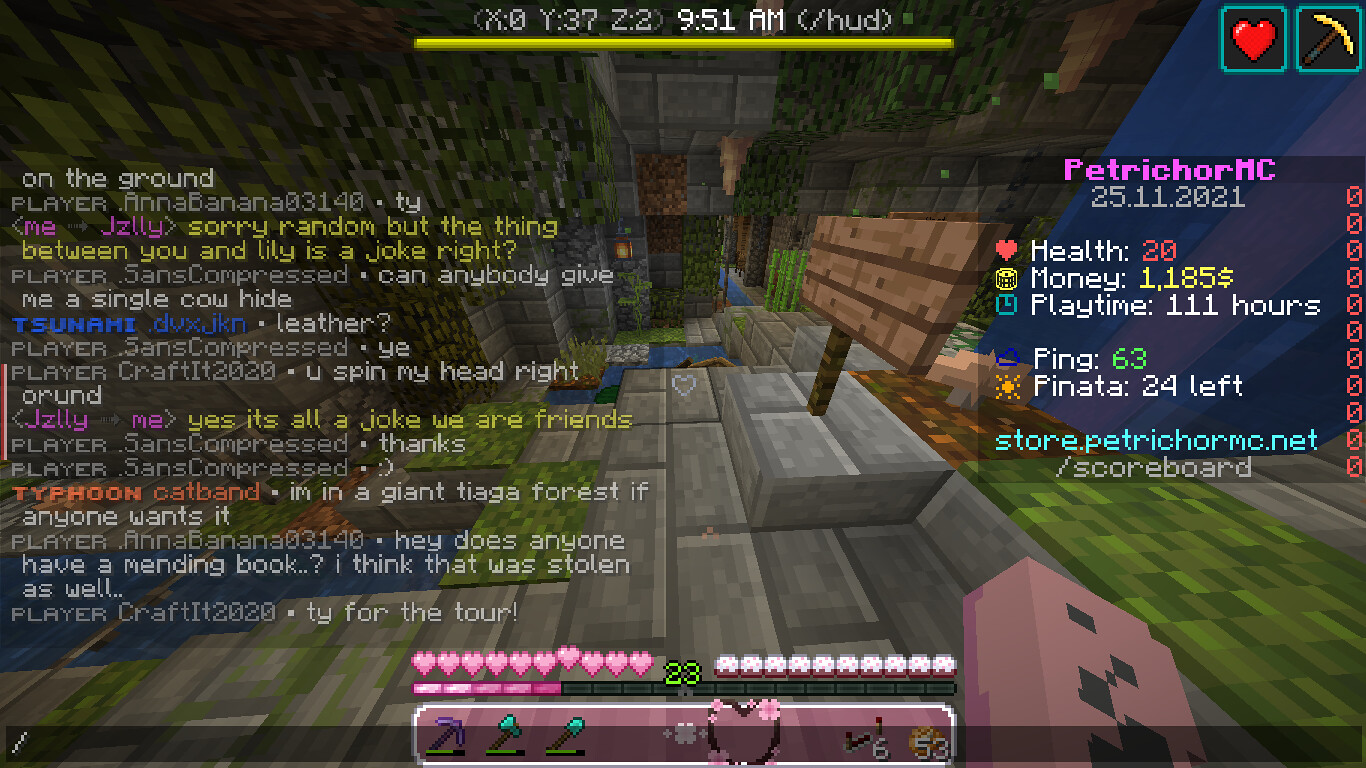The image is a detailed screenshot from a video game resembling Minecraft due to its distinct pixelated graphics. The entire left-hand side of the screen is dominated by a chat box, displaying a constant stream of messages. Below this, at the bottom, there's a user interface featuring a grid of 10 white hearts, likely representing the player’s health, and a row of various pixelated tools including a pickaxe, an axe, and a shovel, characteristic of Minecraft gameplay. Additional unidentified objects are also present. The upper right corner of the screen contains essential game metrics such as health, money, and playtime, with a counter indicating "24 pinatas left" accompanied by a small icon, and the URL of a website. The background showcases green grass terrain, maintaining the blocky, squared aesthetic. A red heart and a yellow wielding tool icon are visible in the top left corner, adding to the overall detailed and immersive game interface.